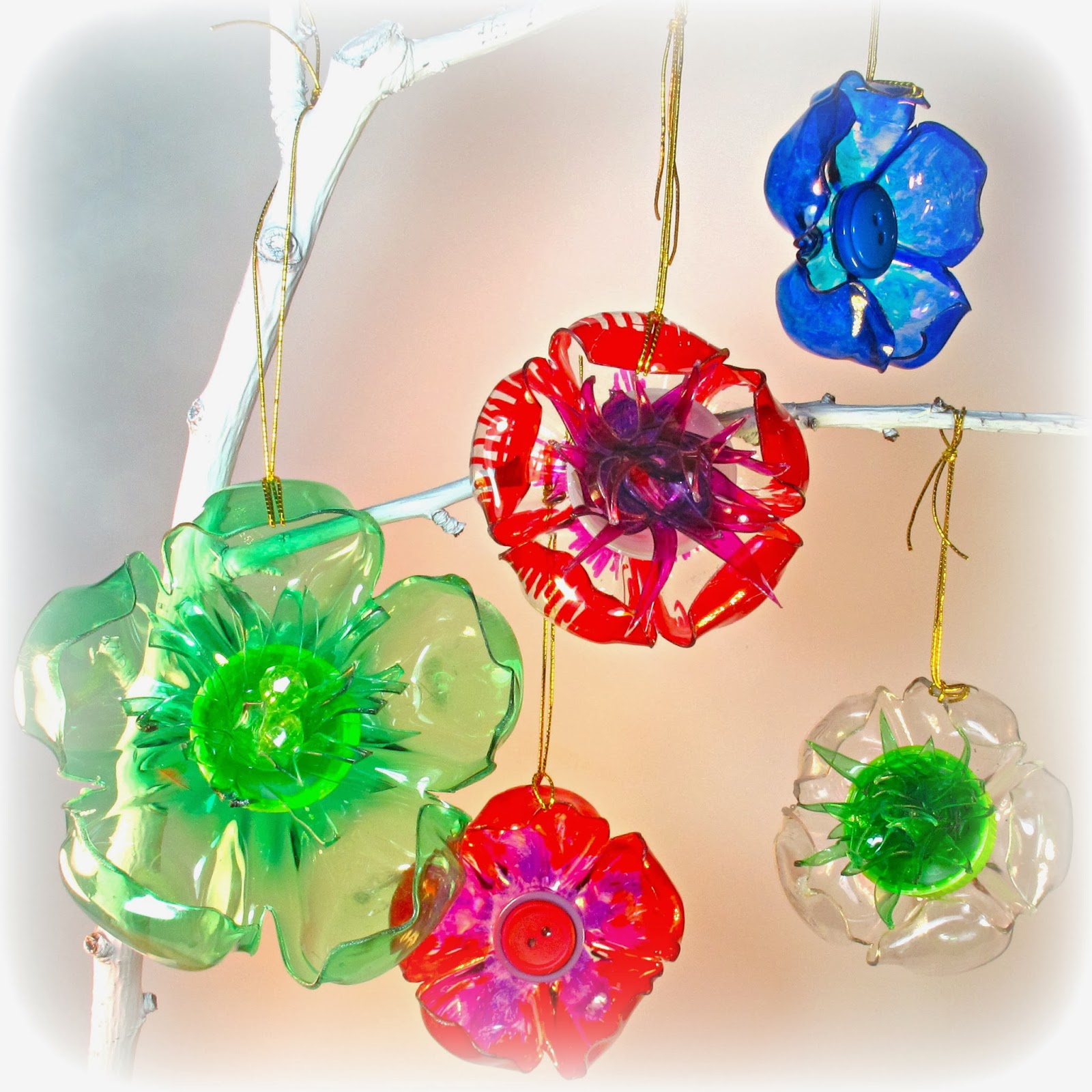This image depicts a detailed drawing of artificial flowers fashioned as Christmas decorations, adorned with golden strings for hanging. A stark white, possibly plastic, tree branch serves as the backdrop, extending from the left with additional smaller branches. The decorations consist of vibrantly colored flowers: a predominantly blue flower with various shades and a blue button-like center positioned at the top right; a fully transparent flower on the right with a dark green and yellow center; a larger greenish flower with transparent petals but more green coloring to the left; below it, a red flower with a purple center and red button at the very bottom; and a central, larger red flower with a purplish center. Each flower, appearing slightly translucent, hangs delicately from the white branches, creating a festive and whimsical atmosphere.